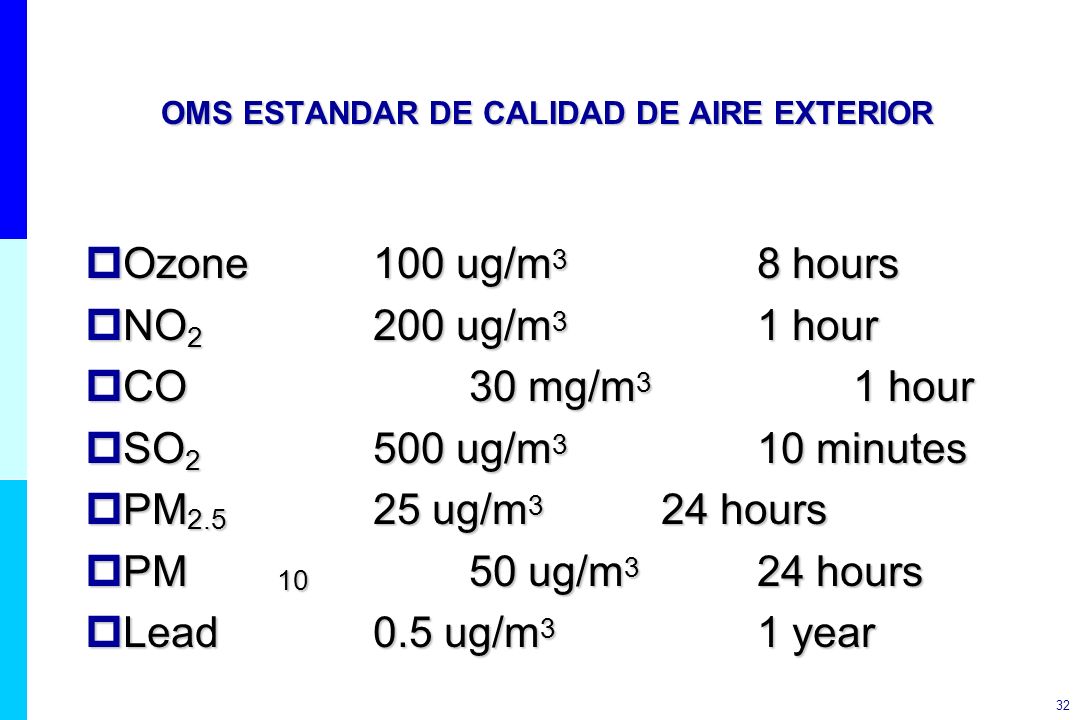The image is a detailed text-only graphic titled "OMS Estandar de Calidad de Air Exterior" in blue font. It contains a table with seven rows and three columns, listing various chemical compounds: ozone (O3), nitrogen dioxide (NO2), carbon monoxide (CO), sulfur dioxide (SO2), particulate matter (PM2.5), PM10, and lead (Pb). Each chemical compound is associated with a unit of measurement (µg/m³ or mg/m³) and a specific time duration. For example, ozone is listed as having a limit of 100 µg/m³ over 8 hours, while CO is limited to 30 mg/m³ over 1 hour. The table includes values such as 200 µg/m³ for NO2 and 0.5 µg/m³ for lead. The alignment is slightly off in the third and sixth rows due to additional spacing issues, with PM10 being misaligned. To the left of these rows are blue checkboxes, none of which are checked. A vertical gradient bar runs along the left side, transitioning from dark to light blue. In the bottom right corner, the small text displays the number 32.